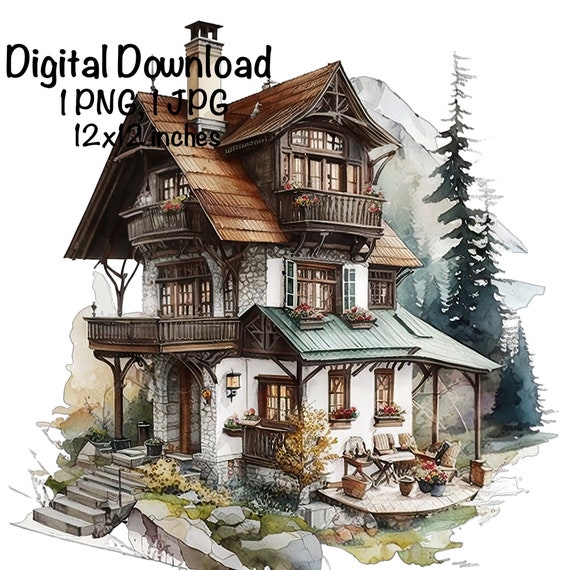This exceptionally detailed image features a charming, old-style country home, potentially set in the United Kingdom. The house stands amidst a forest backdrop, where evergreen trees and expansive grassy areas enhance its quaint and cozy ambiance.

The home is a striking three-story structure, primarily white, featuring an angular design. It boasts a green tin roof on the lower level and two gable-style roofs with brown cedar shingles on the upper level. At the center, a white stone chimney rises elegantly. 

The ground floor's gray stone steps lead up to the entryway porch, which is sheltered by the balcony above and flanked by support beams. Wall-mounted external lights are placed on the right side of the entryway. The patio deck, covered by a green awning, is adorned with a multitude of potted plants and outdoor furniture, including tables and chairs, making it an inviting space for relaxation.

The second floor has four French doors opening onto a balcony that also serves as a roof for the porch below. The balcony is furnished with window boxes and planters overflowing with greenery. On this level, there are flower boxes sitting outside the windows on the tin roof, adding a splash of color.

The third floor’s attic area, characterized by an inverted V-shaped roof, features two additional, smaller balconies on the left and right sides, ideal for standing and taking in the view. The house has a picturesque appearance with these multiple outdoor spaces.

In the upper left corner of the image, partially legible dark lettering on a white background reads, “digital download, 1 PNG, 1 JPG, 12 by 12 inches,” indicating that the image might be a digital download, possibly a drawing or painting. The house's serene setting and meticulous design elements create a timeless and inviting scene.